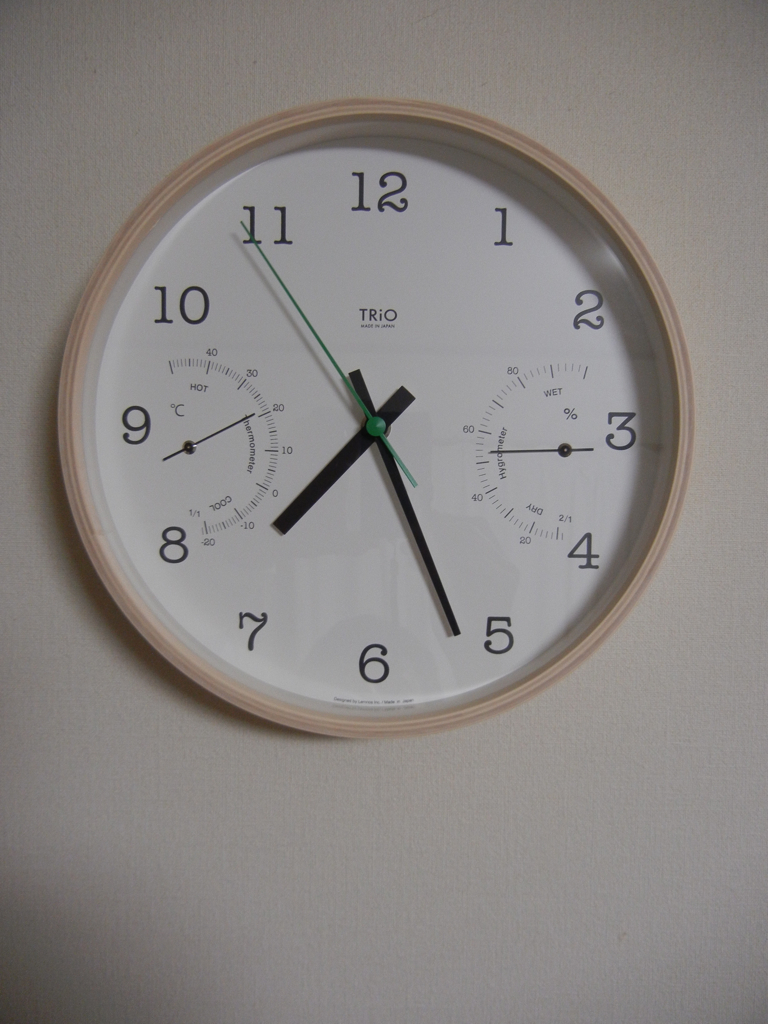This photograph captures a circular clock mounted on a grey wall, which appears to be made of gyprock or weatherboard. The clock features a natural-toned wooden rim that is a blend of brown, yellow, and orange hues. The bright white clock face is adorned with simple Arabic numerals for the hours, eschewing Roman numerals for clear, numeric digits. Displaying the brand name "Trio" in black font near the center, the clock is showing the time as 7:26 and 54 seconds, with the minute hand between the 5 and 6, and the green, thin second hand pointing near 11. The clock’s black rectangular hour and minute hands complement its design.

On either side of the clock face, additional dials provide essential information: the left dial indicates the temperature, currently a bit higher than 20 degrees Celsius, while the right dial displays the humidity level, slightly above 50%. The black hands on these dials add to the clock's detailed functionality. This clock harmonizes aesthetic appeal with practical features, making it a striking yet useful household item.